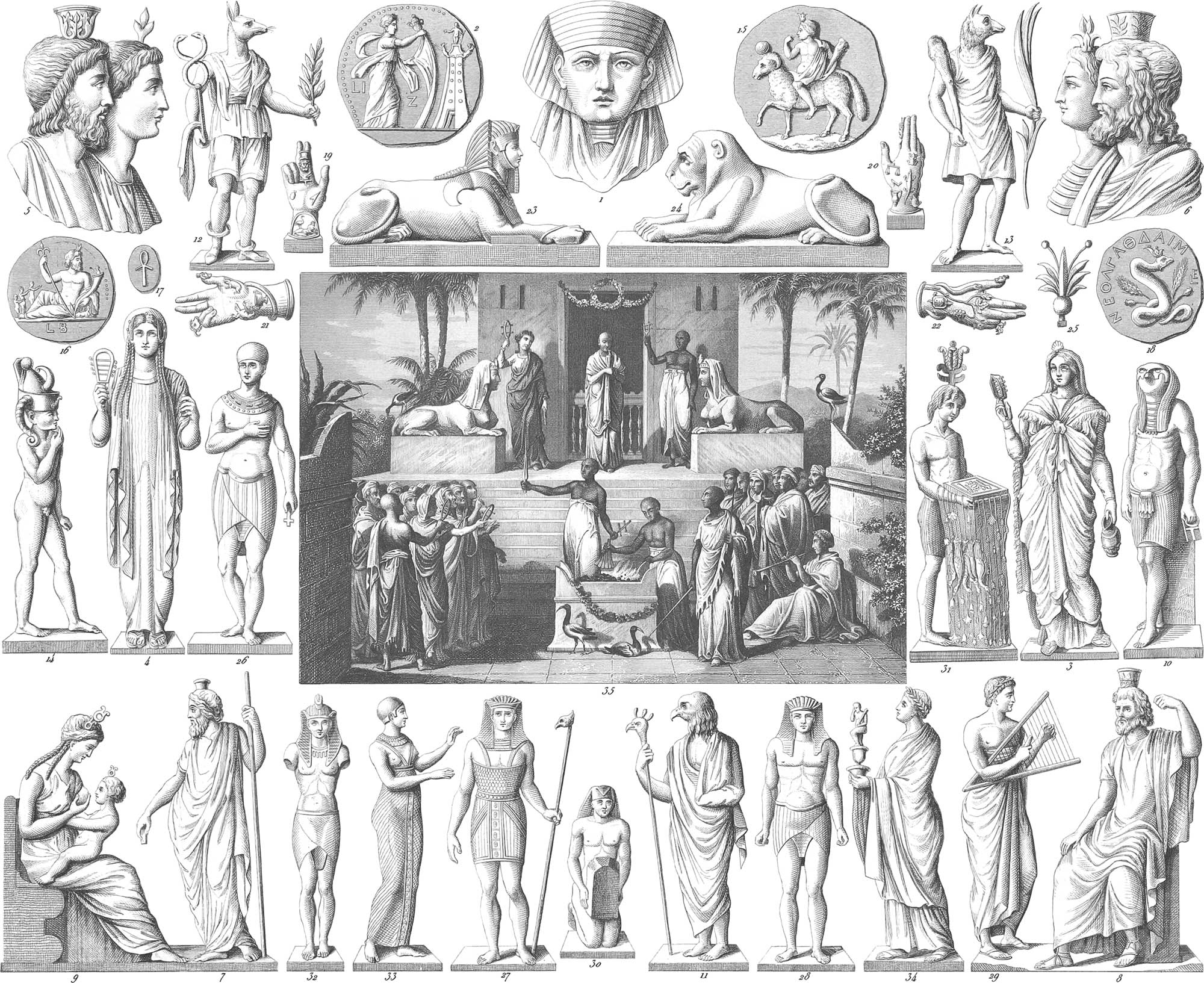The image is a detailed, black-and-white illustration featuring an array of ancient statuary and designs. Central to the illustration is a scene that appears to depict a shrine or altar, flanked by two sphinxes with lion bodies and human heads. This shrine is further populated by a small crowd of figures on both the left and right sides. Surrounding this central scene are meticulously drawn illustrations of various statues, coins, and other artistic designs from ancient Hellenic and Egyptian cultures. The overall composition is structured in three distinct rows, populated with around 40 characters, including figures reminiscent of pharaohs and other notable historical characters. The top row notably features lion-like figures, and the image appears to be rendered either as a pencil drawing or digitally, with the high level of detail suggesting careful craftsmanship.